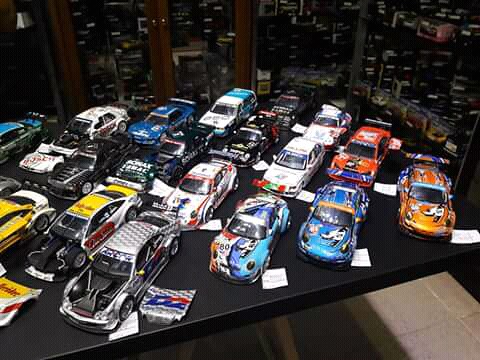The photograph captures a visually striking scene of several colorful model race cars arranged on a black table. The intense flash highlights each car's unique vibrant paintwork, marked with racing numbers. The cars, approximately seven to eight inches long, are all oriented diagonally towards the bottom left of the image, each with a small white piece of paper placed beside the front left tire. The setting appears to be indoors, surrounded by large windows that reveal a high-up cityscape in the background, suggesting that the table is situated on an elevated platform. Many of the model cars display signs of damage, such as crumpled bumpers, adding to their authenticity as racing vehicles. The precise number is unclear, but there are at least a dozen of these intricately detailed models, creating an intriguing and vibrant tableau.